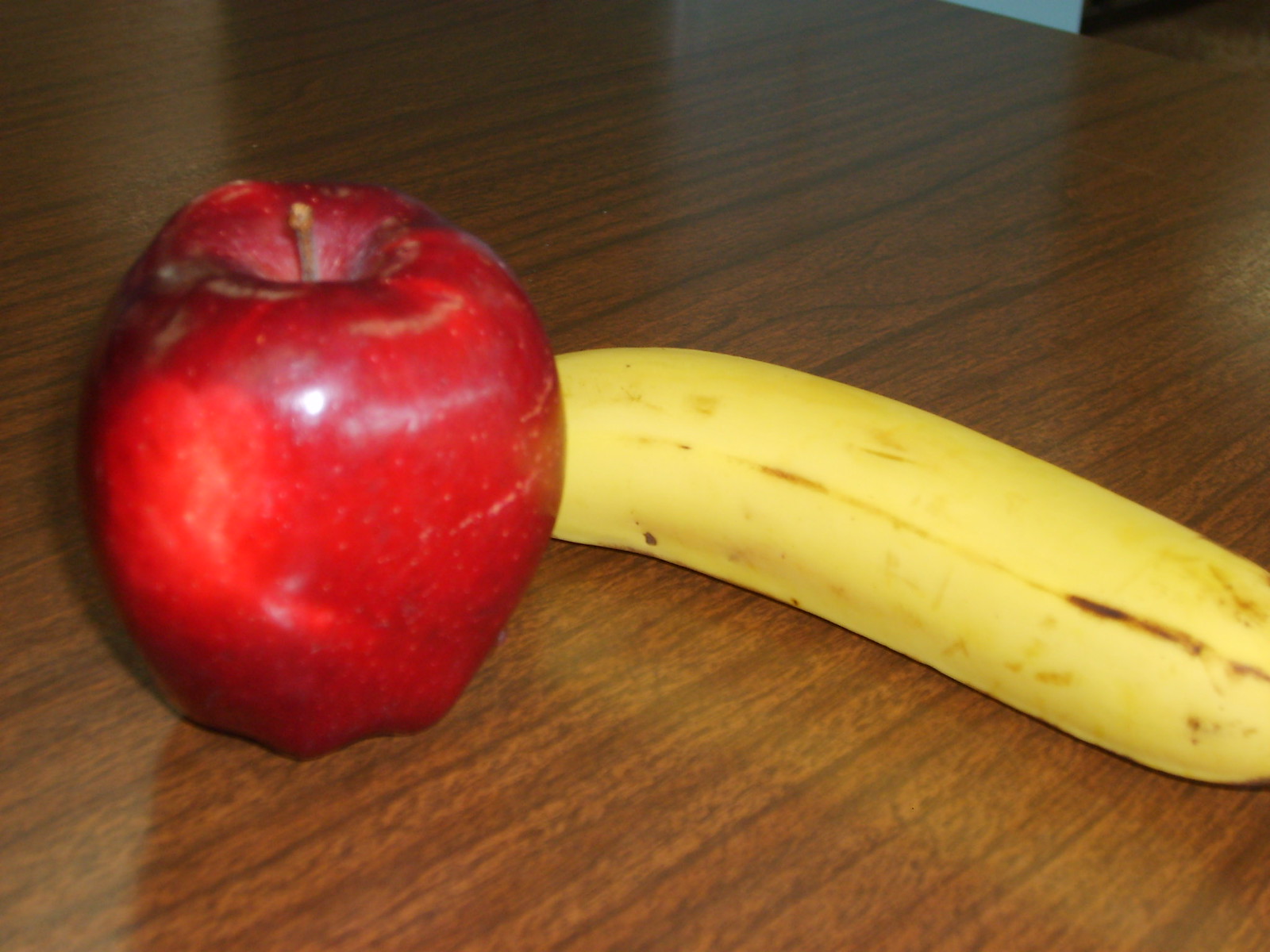A vibrant display of fruit rests on a dark brown wooden surface, characterized by its richly textured grain and scattered darker spots, suggesting it may be a hardwood table or floor. The surface glistens with a few reflective patches, most noticeably on the left and right center, adding depth to the image.

In the foreground on the left, a shiny red apple takes prominence. The apple's glossy skin bears horizontal reflections from overhead light, a testament to its freshness. A slightly rotting brown stem pokes from the top, surrounded by a hint of whitish discoloration. The apple's surface also shows a small crater and a white spot, possibly due to wear or reflecting light.

Behind the apple, a yellow banana curves gracefully across the image, its tip hidden from view behind the apple. The banana's peel is dotted with a few brown spots, indicative of ripeness, but not overly so. It rests comfortably on the wooden surface, extending out of the frame on the right, completing this simple yet vivid portrayal of everyday fruit.